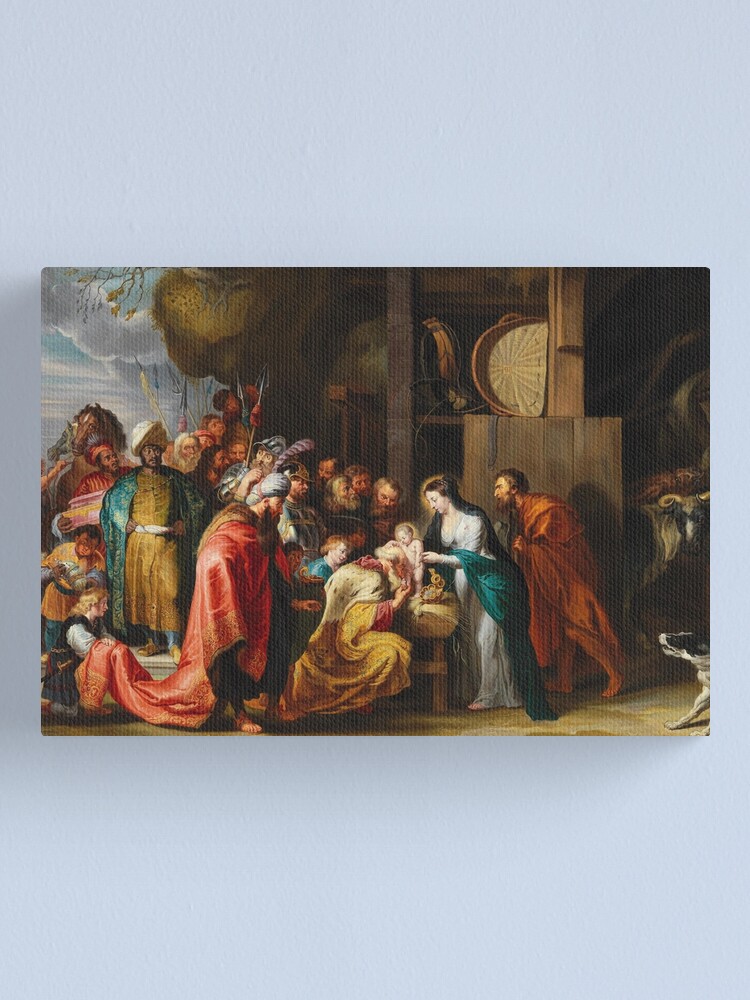The image features a pale blue digital background with a photograph of an old Renaissance-style painting positioned sideways. This painting illustrates a biblical scene, likely the Adoration of the Magi, set in a manger. Central to the image is the Christ child, glowing, cradled by the Virgin Mary, who also has a faint halo. Joseph stands nearby. Surrounding them are numerous figures arching and reaching to see the baby, including three elegantly robed men with turbans adorned with feathers, presumably the Magi. These men are depicted kneeling in front of the infant Jesus. On the lower right, a dog is visible, adding to the scene's richness. The background resembles a barn, complete with a cow, and it opens to a sky filled with clouds. The painting's religious significance is highlighted by the reverence and adoration shown by the figures present.